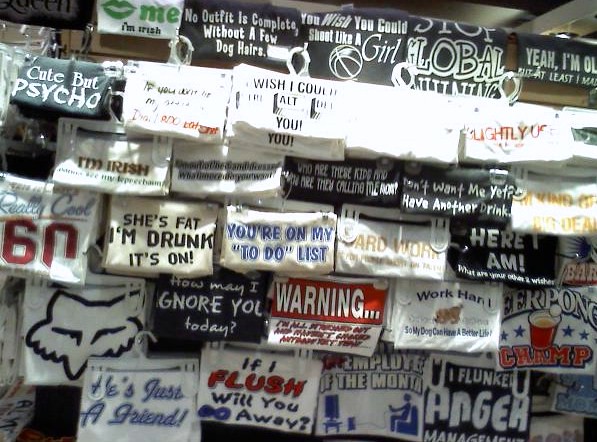This photograph depicts a somewhat blurry collection of t-shirts displayed in what appears to be a store setting, possibly in a bustling area like Venice Beach or Santa Monica. The t-shirts each showcase various humorous, witty, and sometimes provocative texts and designs, making for a diverse assortment. Notable phrases across the shirts include "Cute but psycho" on a green background, "Wish I could alt you" on white, "I'm Irish" printed twice on white backgrounds with green text, and "She's fat I'm drunk it's on" in black text on white. Additional slogans such as "You're on my to-do list," "If I flush will you go away," and "I flunked anger management" in white text on black, add to the playful and irreverent nature of the collection. Some shirts also feature unique graphics, such as a Fox Racing logo, and varied themes with texts like "Stop global warming," "Work hard so my dog can have a better life," and "Beer pong champ" showcasing a red cup and ball design. The eclectic collection speaks to a casual and humorous fashion trend, aimed at attracting attention and eliciting laughs.